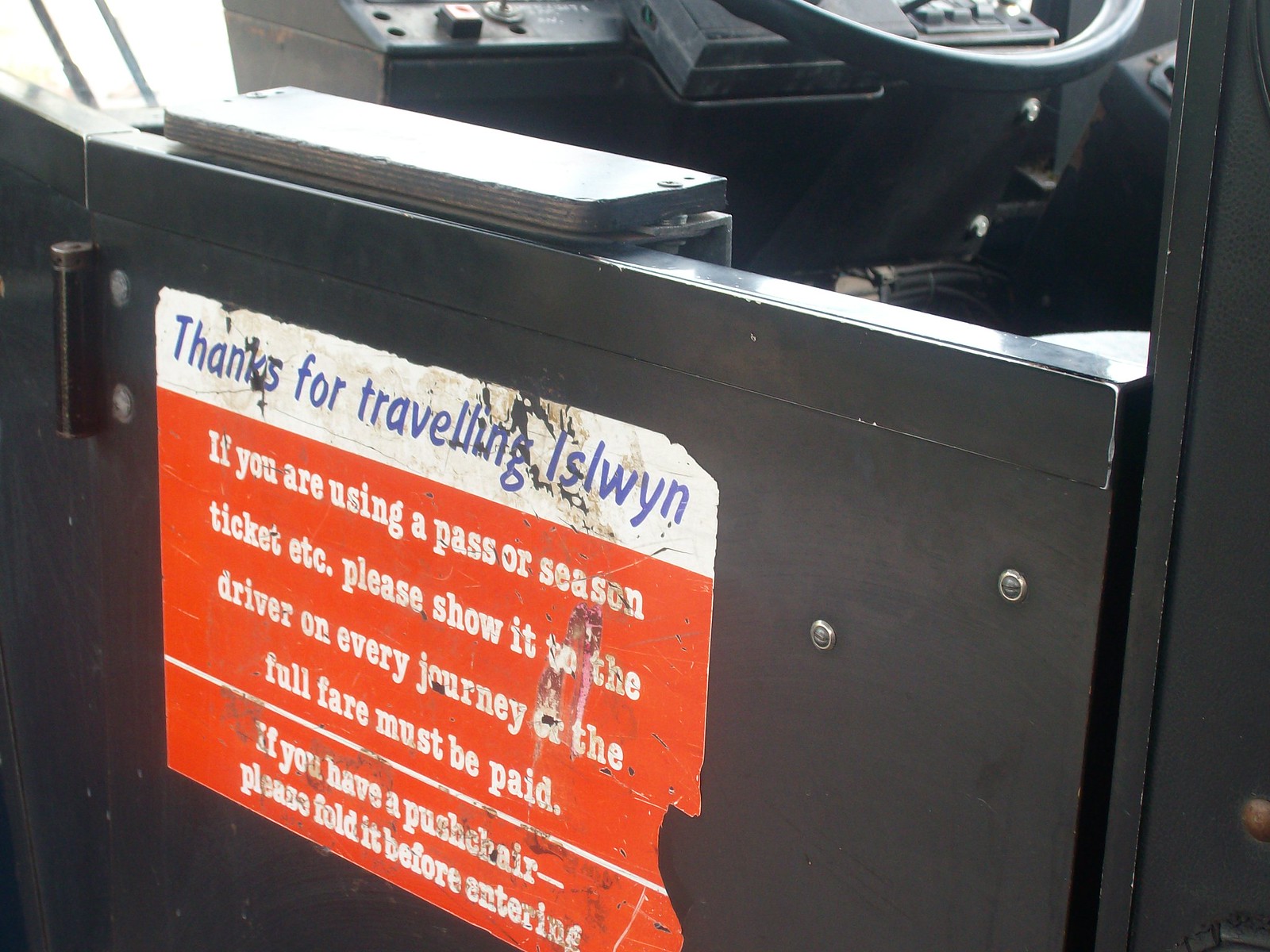The image depicts a worn-out sign affixed to a black swinging metal door next to the driver's cabin of a bus. The door shows signs of wear and tear, with the sticker being notably beat-up and peeling. The sticker, predominantly orange with white text and a white banner at the top, is partially unreadable due to its age and condition. The banner has blue text that reads, "Thanks for Traveling with ISLWYN." The instructions on the sign inform passengers to show their pass or season ticket to the driver on every journey, and to ensure full fare payment. Additionally, it advises passengers with pushchairs to fold them before entering. In the background, the bottom part of the driver’s cabin and some control switches and knobs can be seen. The image captures the practical signage meant to guide passengers as they board the bus.